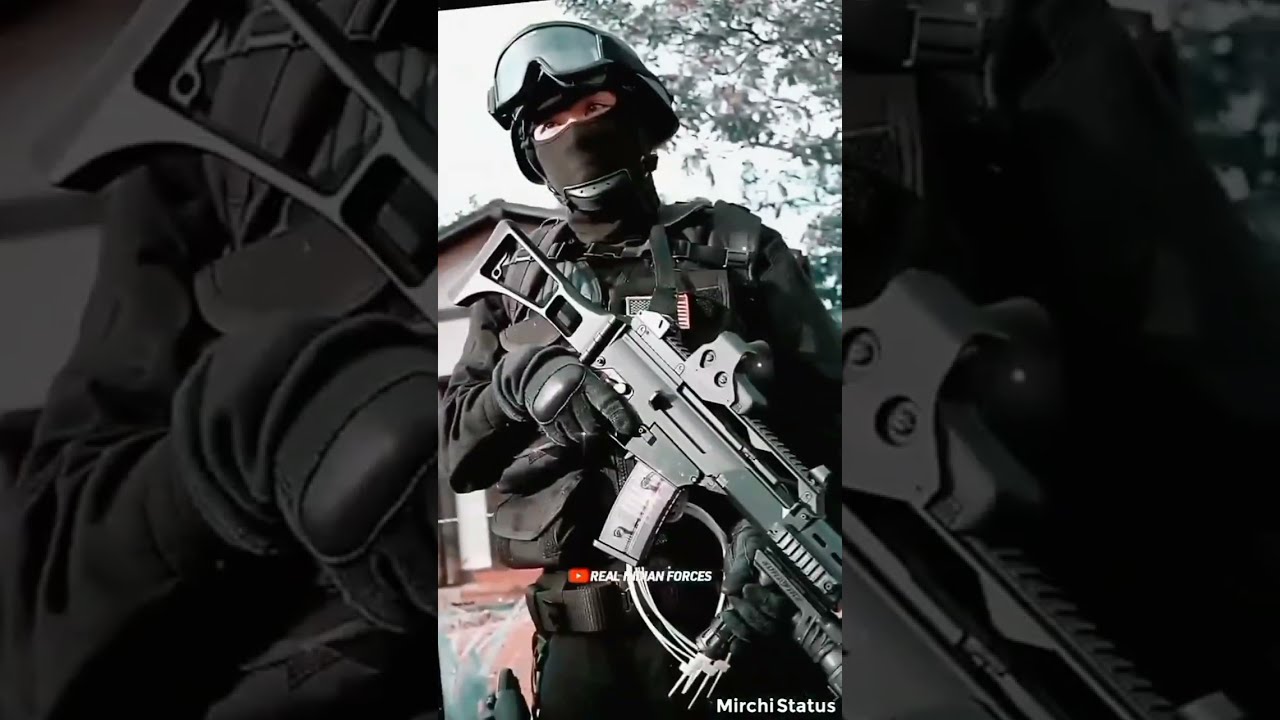The image is a vertically oriented, full-color photograph divided into three panels, forming one cohesive image. The central, highlighted panel prominently features a person dressed in military or riot gear, standing with an assault rifle held at a downward angle with their finger off the trigger. The rifle is equipped with a sight on the top rail. The individual is clad entirely in black, including a tactical vest with extra ammunition and black gloves. The person is wearing a black helmet with ski goggles perched on top and a black balaclava covering their face, leaving only a small slit open for the eyes. A chin strap from the helmet is visible beneath the face covering. 

The left and right panels are translucent, zoomed-in close-ups of the center image, providing an enlarged view but obscured by the central overlay. In the background of the central panel, there is an overhanging tree on the right and a structure resembling a house or shed with a peaked roof on the left. Notably, there is an American flag patch on the individual’s gear. The image also features a red button icon indicative of a video play feature, labeled with "Real Maxim Forces," and the words "Mirchi status" in the lower right-hand corner.